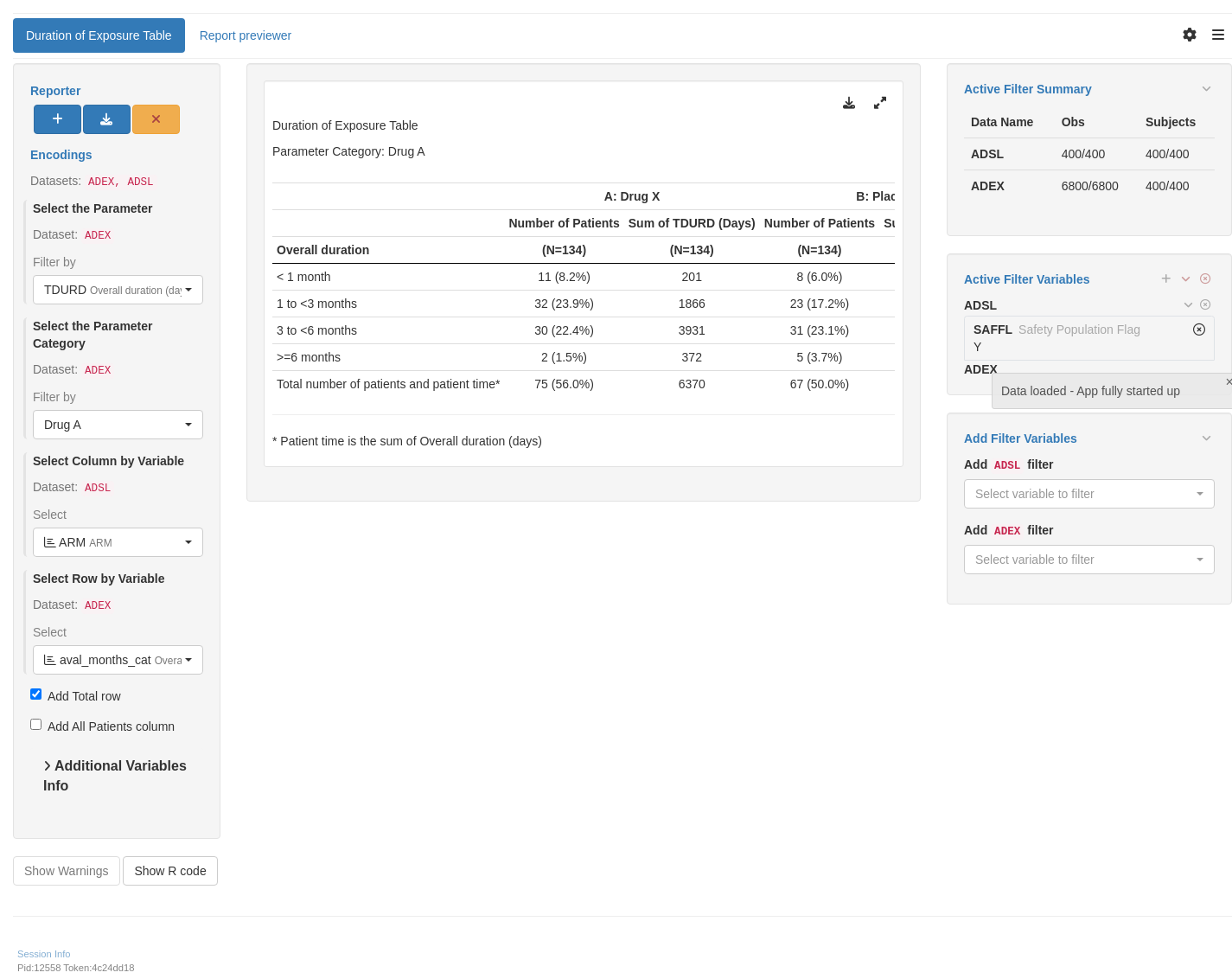This image is a screenshot of a data table from a website, specifically titled “Duration of Exposure Table.” The table is central to the screenshot and displays detailed information categorized around a parameter for different drugs: Drug A and Drug X. The table seems partially obscured but provides significant detail where visible.

The columns are labeled to represent various metrics for the duration of exposure in patients, segmented into multiple time frames: less than a month, one to less than three months, three to less than six months, more than or equal to six months. Each segment details the total number of patients involved, listed under the title "Number of Patients” and another column titled "Sum of T, D, U, R, in parentheses, indicated in days."

For Drug A, the overall duration of patient exposure is broken down as follows: 11 patients with less than a month of exposure, 32 patients between one to less than three months, 32 patients from three to less than six months, and 75 patients with more than or equal to six months of exposure. 

Another similar set of data is provided, though the exact contextual framework is not entirely clear, as some of the data columns are partially visible. The numbers in the next column seem to indicate further patient-related metrics such as:
- 201, 18, 66, 39, 31, 372, 63, 70 for Drug X
- Another patient count of 8, 23, 31, 5, and 67 

In conclusion, this elaborate table captures the exposure duration across different patient categories, providing insights into the data frequency and exposure timings for Drug A and Drug X.